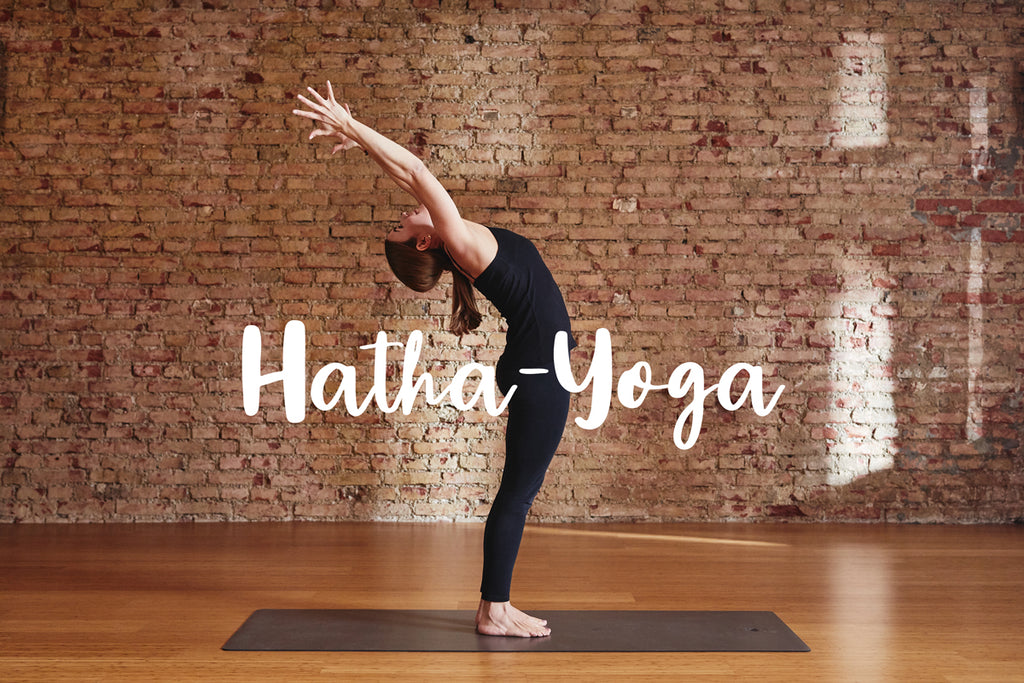A woman stands barefoot on a brown yoga mat in an indoor studio, performing a Hatha Yoga pose. Her back is arched, and her head tilts back with her hands extended behind her head. She has long brown hair pulled into a ponytail that cascades towards her lower back. She is dressed in a black tank top and black yoga pants. The studio features a tall, rough brick wall that seems repurposed from an older structure, and a smooth, well-maintained wooden floor. Sunlight filters through unseen windows, casting reflections and shadows on the floor and brick wall. Superimposed across the image in white lettering is the phrase "Hatha Yoga."